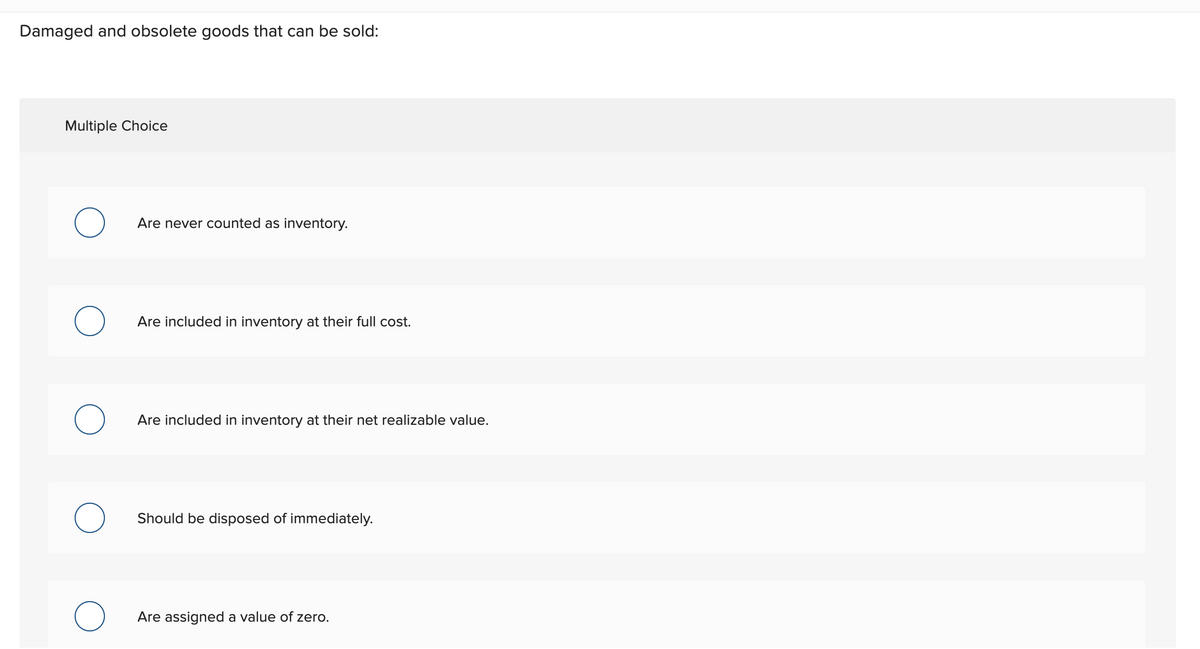In the image, the background is plain white. Positioned at the top left in bold black font, there is a heading that reads "Damaged and Obsolete Goods that Can Be Sold." Below this heading, in a slightly grayer font, it states all at the top left, “Multiple Choice,” followed by five intervals, each containing options for selection. 

Each interval consists of a small, white, square-shaped option button outlined in black, with a corresponding circle inside, also outlined in black. Adjacent to each of these buttons are the following descriptive options:

1. The first line reads, "are never counted as inventory."
2. The second line states, "are included in inventory at their full cost."
3. The third line says, "are included in inventory at their net realizable value."
4. The fourth line specifies, "should be disposed of immediately."
5. The fifth line declares, "are assigned a value of zero."

The image appears to cut off at the bottom, with the final interval's square not being completely visible.